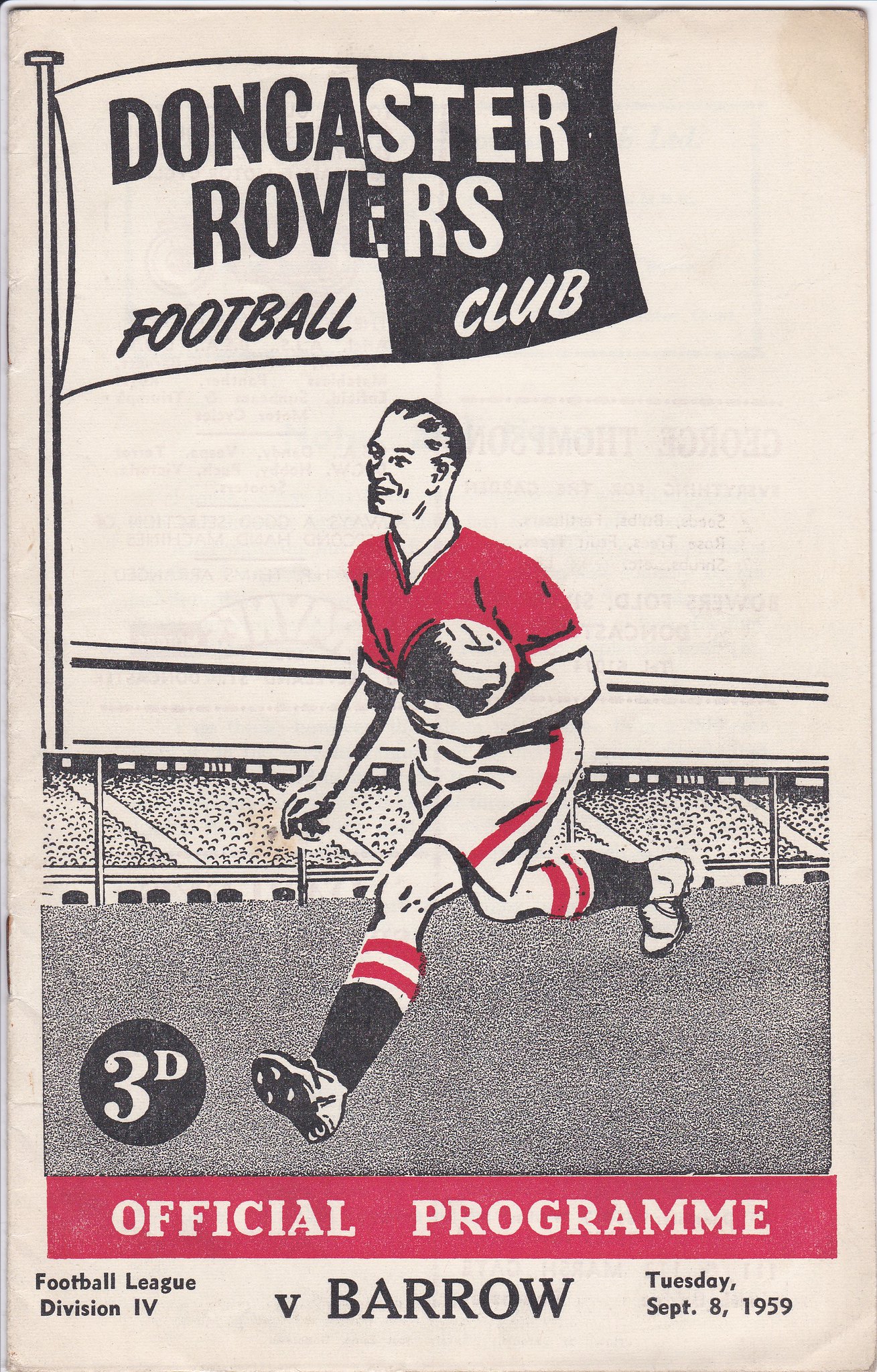The image is an old-school cover for the official program of Doncaster Rovers Football Club, dated Tuesday, September 8, 1959, for a match against Barrow in Football League Division Four. The cover features a cartoon drawing of a man running left to right across a football field, holding a football. He is depicted wearing a red jersey with white collars and cuffs, white shorts with red lines on the sides, and black socks with red and white stripes at the top. A stadium filled with spectators serves as the backdrop.

The top section of the cover displays a flag—half white, half black—emblazoned with "Doncaster Rovers Football Club" in alternating black and white print. Notably, the letters D-O-N-G-A and R-O-V in ‘football’ are in black, while S-T-E-R-S in ‘club’ are in white.

The cover has a portrait orientation with dimensions taller than wide, including a thin white border on the left and top edges. Two staples are visible on the left side, indicating it is a magazine-style publication. The paper has a yellowed, aged appearance. 

In the lower left-hand corner of the field illustration, there is a small black circle containing the white text "3D." Below the image is a red rectangular banner with white text that reads "Official Program," and at the very bottom, it states "Football League Division Four" with details of the match against Barrow.